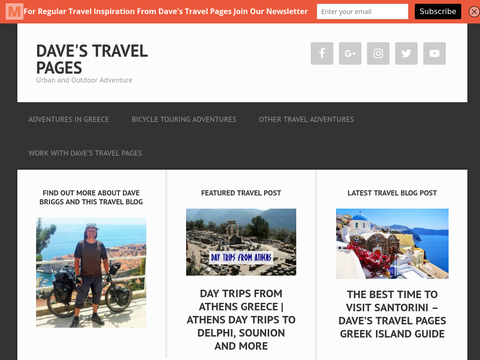**Caption:**

The image showcases the homepage of "Dave's Travel Pages," a travel blog. In the top left corner, the blog's name, "Dave's Travel Pages," is prominently displayed in white text on a gray background. Below this, the tagline "Urban Outdoor Adventure" is written in light gray. At the very top of the webpage, a red header bar invites users to join the newsletter for "regular travel inspiration from Dave's Travel Pages," featuring an empty dialogue box for email entry with placeholder text. A black hyperlink button labeled "Subscribe" in white text is located to the right, next to a semi-transparent, greyscale "X" symbol.

Directly below the blog name, there are icons for social media platforms: Facebook, Google Plus, Instagram, Twitter, and YouTube, all in light gray with white symbols. The main part of the page is divided into two sections: the left side features a black background with three highlighted categories—Adventures in Greece, Bicycle Touring Adventures, and Other Travel Adventures. Below this is another header encouraging users to "Work with Dave's Travel Pages."

The lower portion of the image includes three article sections. On the left, a man sits with his bike among palm trees, serving as a link to "Find out more about Dave Briggs and his travel blog." The middle section highlights a featured travel post, likely showcasing day trips from Athens, Greece, including Delphi and Sounio. On the right, a recent travel blog post about the Greek Islands is shown, with a serene image of water and a title that reads, "The Best Time to Visit Santorini, Dave's Travel Pages Greek Island Guide."